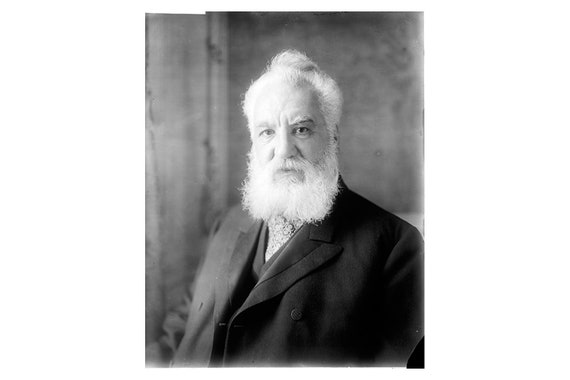This detailed black-and-white photograph depicts an elderly man with white hair, a thick white beard, and a mustache. His hair is receding slightly at the front and puffs up in the middle, almost forming a small bun. He has white, scrunched eyebrows with two vertical lines between them, giving him a somewhat stern expression. He is dressed in a dark suit, possibly with an overcoat, and a lighter tie or similar neckwear. The image captures him from the chest up, with his body turned slightly to the left while his head faces forward. The background features a light gray wall with variations in shading and what appears to be a corner, as well as a small black triangle in the bottom right corner, the origin of which is unclear.